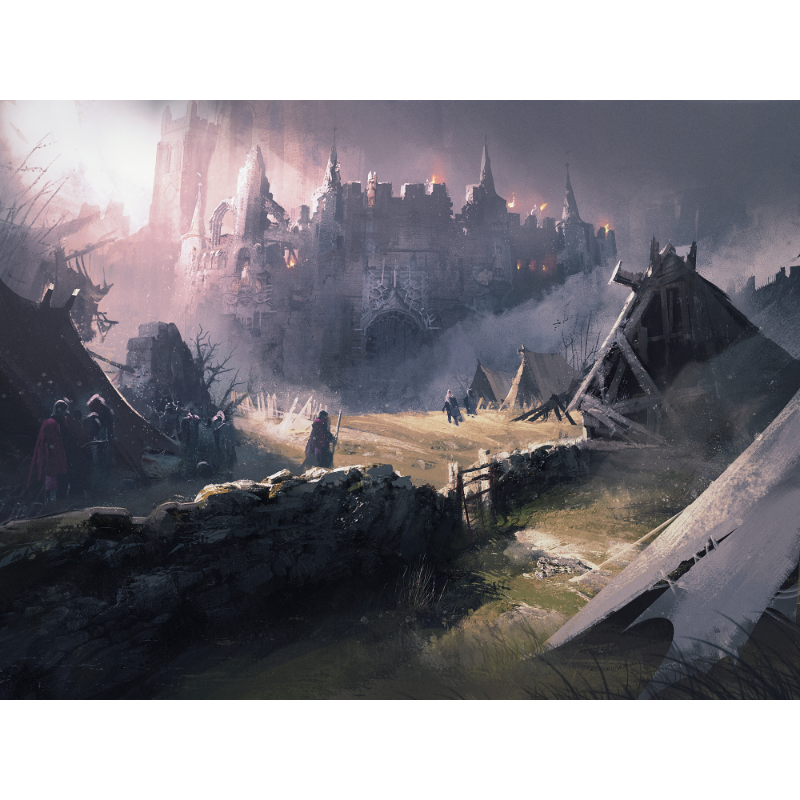In the foreground of this dark and gloomy scene, amidst grassy terrain, there are a couple of teepees with people walking around them, possibly dressed in armor. Nearby, dilapidated wooden structures and metal debris suggest a history of neglect. On the left side, a rock fence with a metal gate extends towards the right, framing the area where some people are huddled. Moving left towards the center, an amber-robed person stands out among others, including one holding a pole.

The background features a foreboding light gray castle with a blue tint, enshrouded in smoke and flames emerging from its top. The castle’s architecture includes sharp points capped with crosses and a large oval arched doorway. The upper left corner of the sky is yellow and hazy, contributing to the ominous atmosphere of the scene. This image, possibly from a video game or painting, conveys a sense of medieval decay and desolation through its detailed and evocative elements.